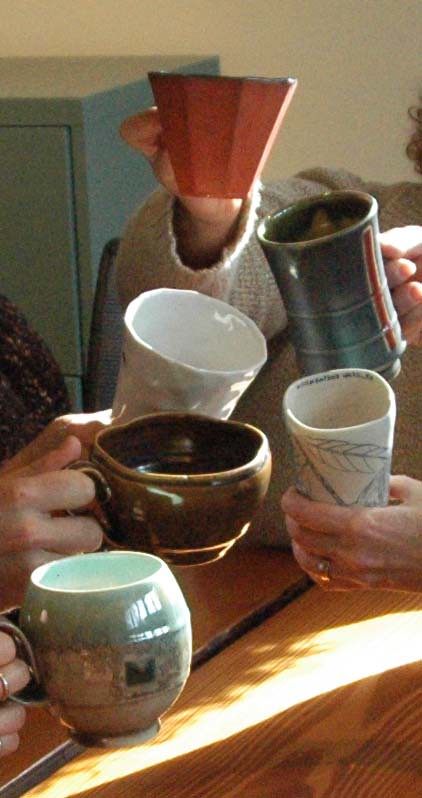This image captures a close-up of several hands, each holding a uniquely styled coffee cup, all gathered over a wooden table in what appears to be a home. Dominating the scene is a woman in a gray long-sleeved sweater, her hand gripping a red cone-shaped, flat-sided cup. To her right, a tall gray cup with a red stripe stands out, alongside another hand adorned with a gold ring, holding a tall, square-shaped white cup decorated with a feather design. On the left side of the group, a short, blue, round, almost ball-shaped cup, a short, unevenly crafted brown cup with a bumpy rim, and a shiny, tall, skinny white ceramic cup can be observed. Completing the scene, a green ceramic mug and another white cup with designs are also held up in a toast. The background features a bluish-green filing cabinet against a white wall bathed in natural daylight, adding to the cozy ambiance of the setting.